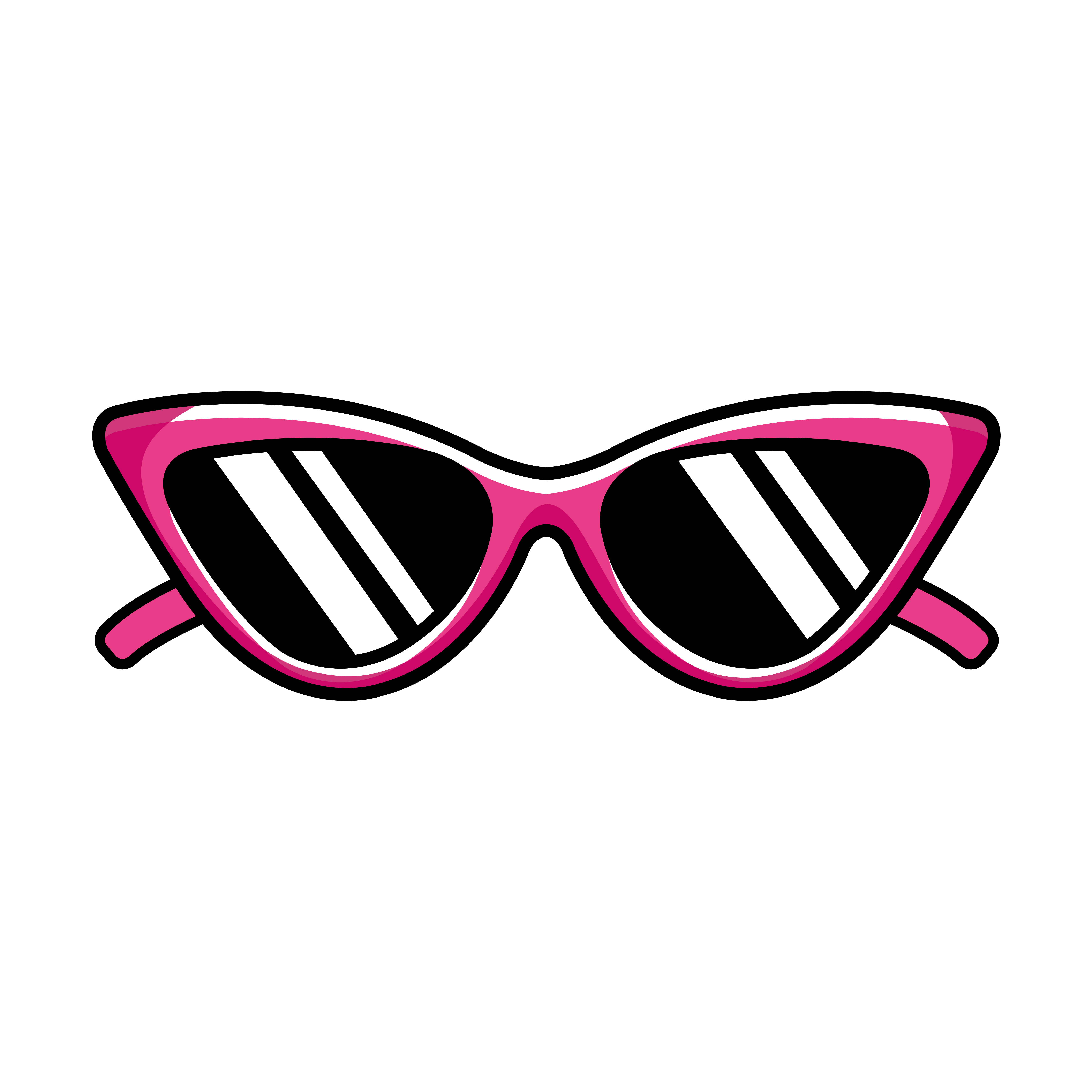The image is a digital illustration of a retro-style pair of cat-eye sunglasses set against a white background, which helps to make the vibrant colors stand out. The frames of the sunglasses are a striking hot pink, with subtle red accents underneath to give a shadow effect and add depth. These frames flair slightly at the upper outer corners to emphasize their cat-eye shape. The lenses are jet black, featuring two diagonal white streaks from the top left to the bottom right of each lens, creating an illusion of reflection and suggesting shininess. A white stripe also runs along the top bridge of the frames, enhancing the reflective appearance. The ear pieces are partially visible, folded up to not detract from the main view of the sunglasses, ensuring that the focus remains on the detailed and colorful design of the frames and lenses.